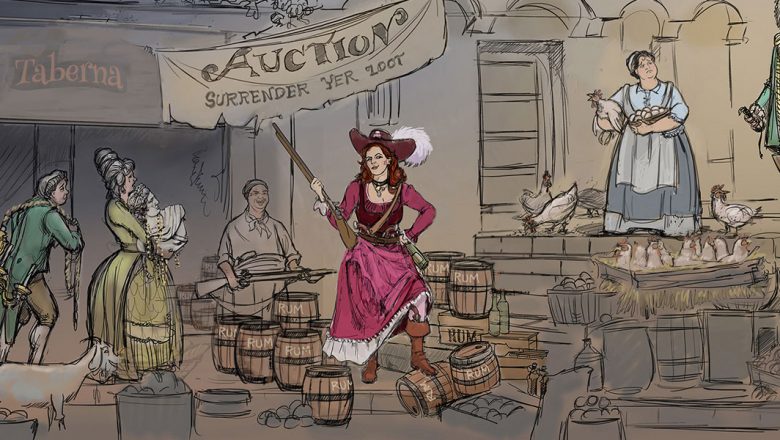The illustration depicts an old Western setting, centered around a lively courtyard scene that seems pulled from a bygone era. A large sign hangs prominently from one of the wooden, weathered buildings, proclaiming "Auction, Surrender Your Loot." The scene is bustling with activity, featuring five women in colorful dresses—purple, blue, green, burgundy—some adorned with hats while others brandish rifles. One woman, reminiscent of an Annie Oakley figure, hitches up her burgundy can-can dress, revealing a pistol in her boot and a shotgun resting on her hip.

The courtyard is animated with various livestock, including chickens that roam freely and a notable goat that adds to the rustic charm. Barrels, presumably filled with liquids, are scattered around, heightening the sense of a bustling market day. One woman in a blue dress stands on a stage, holding two chickens, with another nestled in a basket of eggs nearby. Her vivid blue attire contrasts with the earthy tones of the setting.

Beside her, a man in old pants and a green jacket wields a sword, maintaining a vigilant stance. The background is filled with shades of gray and brown, reinforcing the Western motif. The detailed textures of the wooden structures, barrels, and the characters' attire contribute to an immersive, well-crafted scene that tells a rich story of a town caught in the throes of an auction day.